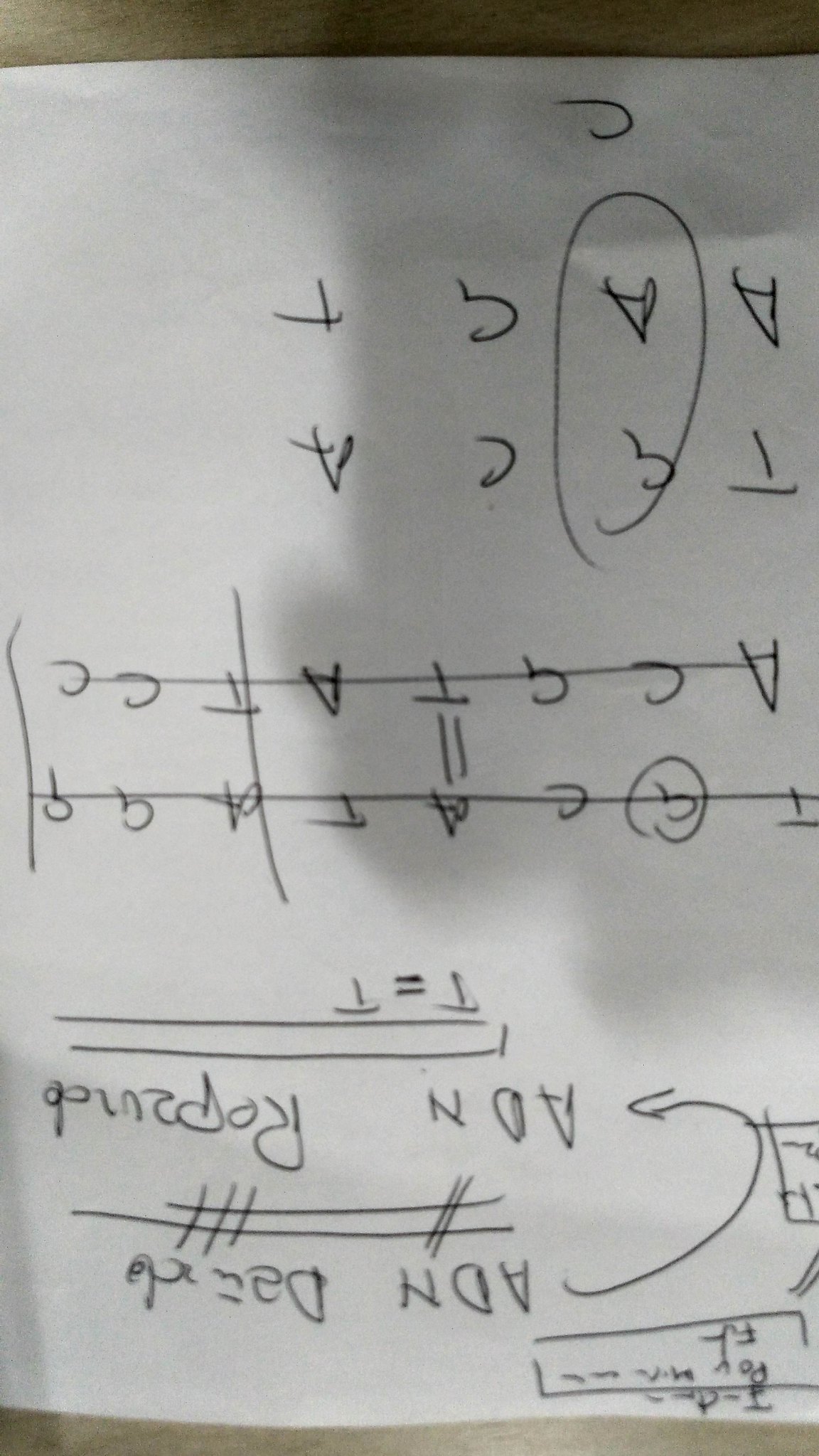### Caption:
Color photo of handwritten notes on DNA sequencing, displayed upside down. The notes are on a piece of paper resting on a table, with a bit of the tabletop visible at the top of the image. The paper details the pairs of amino acids in DNA strands.

The text begins with "ADN," followed by partially illegible words and arrows indicating a sequence or process. T equals T is noted, alongside drawings of DNA chains. Here's what's visible:

1. An 'A' paired with a 'T'
2. A 'C' paired with a 'G'
3. A 'G' (circled) paired with a 'C'
4. A 'T' paired with an 'A'

The bottom of the page (top of the image) shows more nucleotide pairs:

1. A 'T' paired with an 'A'
2. A 'G' paired with an 'A' (circled)
3. A 'C' paired with a 'G'
4. An 'A' paired with a 'T'

Underneath the circled 'G' and 'A', there's a 'C' written. The notes highlight basic DNA coding with adenine (A), thymine (T), cytosine (C), and guanine (G). The handwriting is in uppercase, though the Gs have an unconventional style, resembling Cs with a downward tail. This document illustrates fundamental DNA sequencing and pairing.